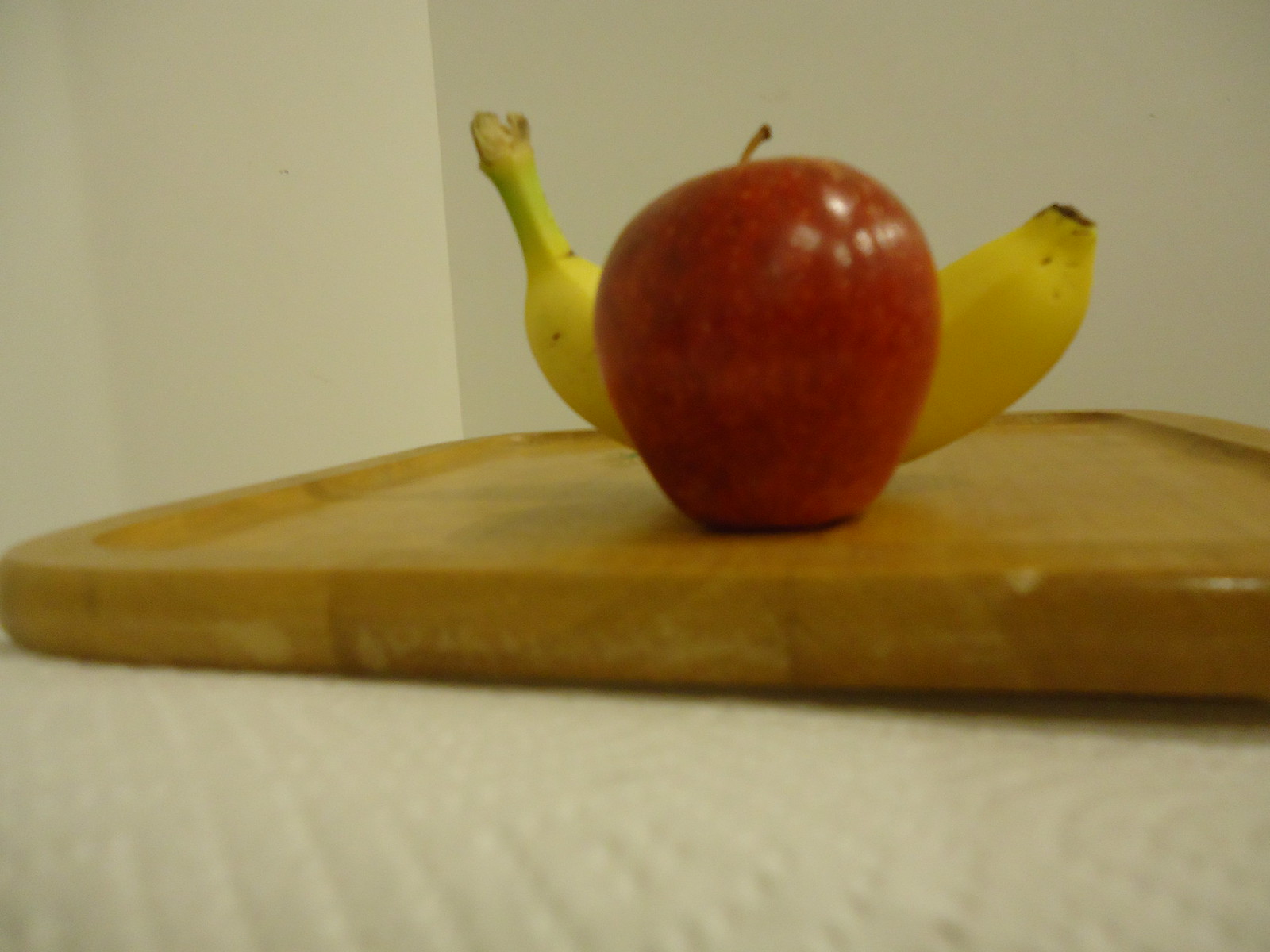In a warmly lit kitchen with soft ivory-beige walls, this photograph captures a humble yet inviting scene. At the forefront, an old, pale wood cutting board tells tales of many culinary adventures with its slightly faded and worn edges. Although the image quality is low and somewhat out of focus, the textures of the cutting board remain defined. Resting atop the cutting board is a shiny red apple and a single banana, both vibrant and ripe, suggesting freshness and readiness to be enjoyed. The apple, with its glossy skin, and the banana, slightly curved, contribute a splash of color to the otherwise neutral-toned surroundings. A layer of paper towel, visible through its perforation marks under the cutting board, adds an informal touch to the setup. Despite the overall blur, the back corner of the room stands out in sharp focus, hinting at a mistaken focus by the photographer. This subtle detail underscores the spontaneous, everyday essence of the captured moment.